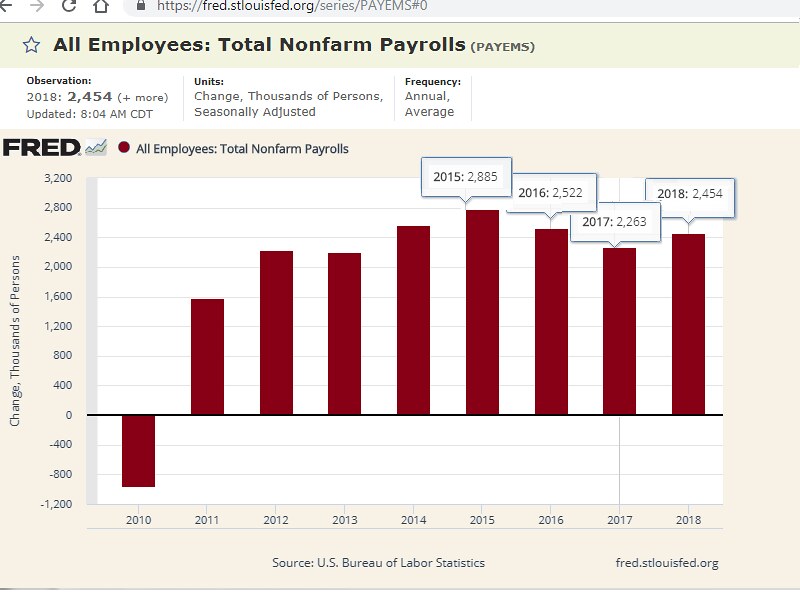The image displays a bar graph titled "All Employees: Total Non-Farm Payrolls," sourced from the US Bureau of Labor Statistics via Fred.StLouisFed.org. The chart spans from the year 2010 to 2018, illustrating the annual average change in thousands of persons, which is seasonally adjusted. On the left vertical axis, it ranges from -1,200 to +3,200. In 2010, the red bar indicates a decline, falling below -800. From 2011 onwards, all bars are positive, surpassing 1,200, with the highest bar in 2015 at 2,885. The 2018 observation is noted as 2,454. A notification at the top of the graph indicates the last update was at 8:04 AM CDT.